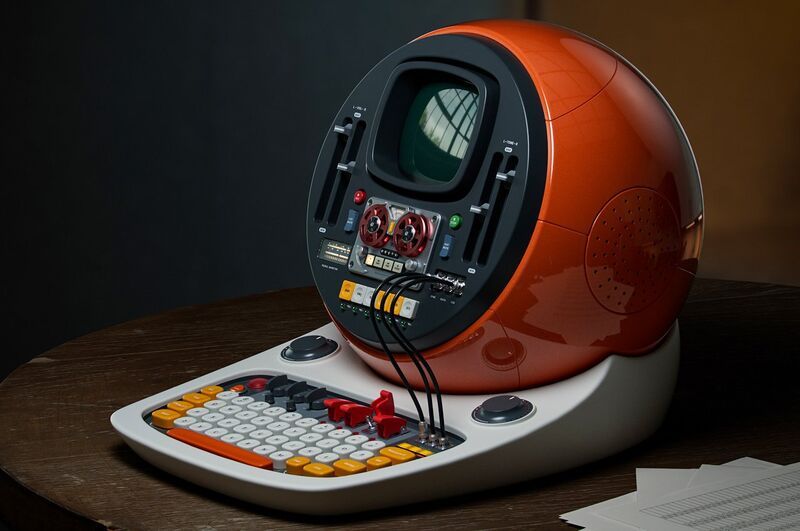The image portrays a highly detailed 3D-rendered, retro-futuristic computer, embracing a design aesthetic from the 1950s vision of future technology. The central feature is an orange, spherical monitor that blends seamlessly with a white keyboard base, creating a unified, compact device. The small, square-shaped screen, embedded in the top part of the orange sphere, is surrounded by various controls. On either side of the monitor, there are two knobs and levers that suggest adjustable functionalities. The front interface consists of a black circular panel equipped with multiple knobs, switches, and an integrated reel-to-reel tape player with orange reels. Beneath the tape player, there are four buttons that illuminate when pressed, and an additional series of buttons, three yellow and three gray. The keyboard itself features predominantly white keys, with some yellow keys interspersed, and a dark orange spacebar. The construction material appears to be plastic, contributing to the retro aesthetic. A set of indentations on the side likely serves as a speaker, enhancing the machine's multi-functional appeal. Some wires connect the main body to the keyboard, completing a vision of a compact, all-in-one retro-futuristic computer system.